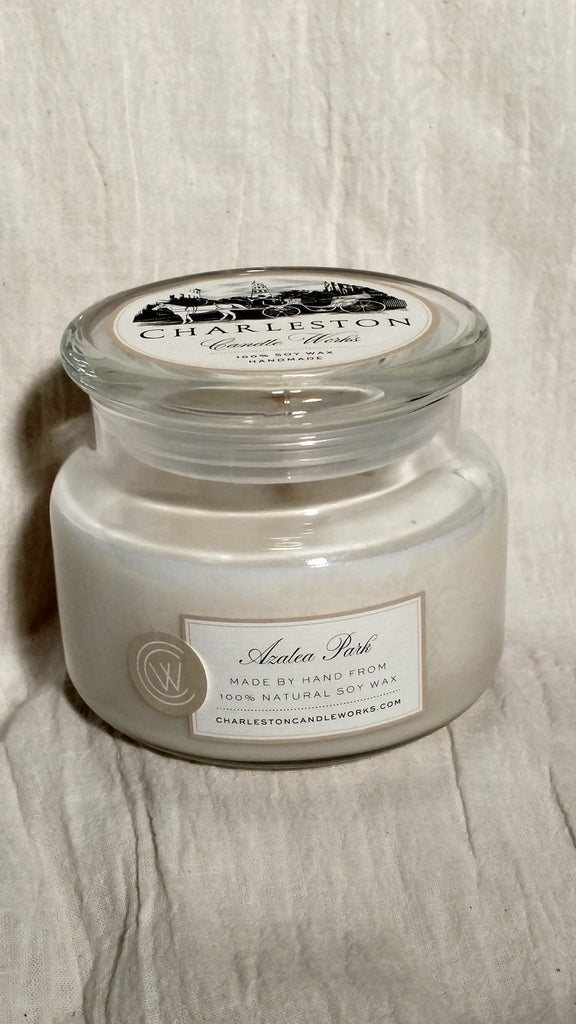The image is a portrait-oriented photograph featuring a close-up of a small, short candle housed in a clear glass jar. The candle itself is white and is set against a wrinkled, light white or grayish fabric background. The top of the jar has a circular, white sticker with a black sketch that appears to depict a horse-drawn coach, alongside the text "Charleston" in black and some cursive text beneath it which is hard to read. Below this cursive text, two lines of small, unreadable text are present as well. 

On the front of the jar is a white label bordered in gray. In the center of this label, in black cursive, it says "Azalea Park." Below this, the label reads, "made by hand from 100% natural soy wax," followed by "charlestoncandleworks.com." There is also a circular emblem on the left side of this label with the initials "CW" inside. The image does not feature any people or additional text aside from the labels on the candle.